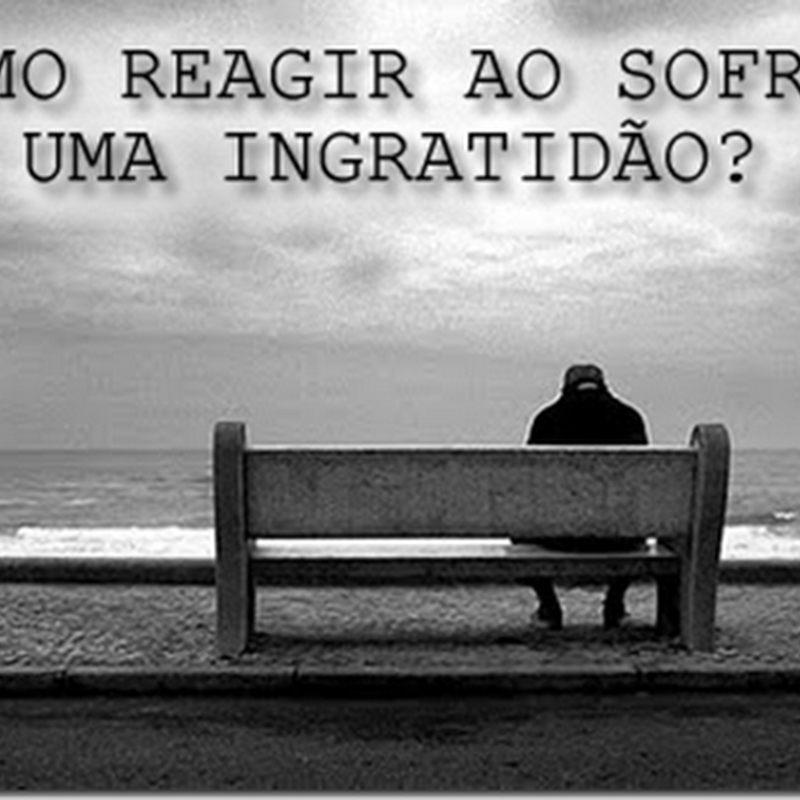The image is a grayscale, vertical rectangular meme of a man sitting on a concrete bench at the beach, looking out at the ocean. The entire scene is rendered in black and white. The man, whose back is mostly visible, wears a dark outfit including a cap, black jacket, black pants, and black shoes. He is seated on one corner of the wide, three-seater bench, with his head down, suggesting a contemplative or sad mood. The bench is positioned on a pavement strip, with a narrow road behind it. In front of the man, the expanse of the sea stretches out to meet the sky, which is dotted with discernible clouds. Thin, black, foreign-language text overlays the clouds, reading "M-O-R-E-A-G-I-R-A-O-S-O-F-R" on the first line and "U-M-A-I-N-G-R-A-T-I-D-A-O?" on the second line, likely offering an inspirational or thoughtful message.